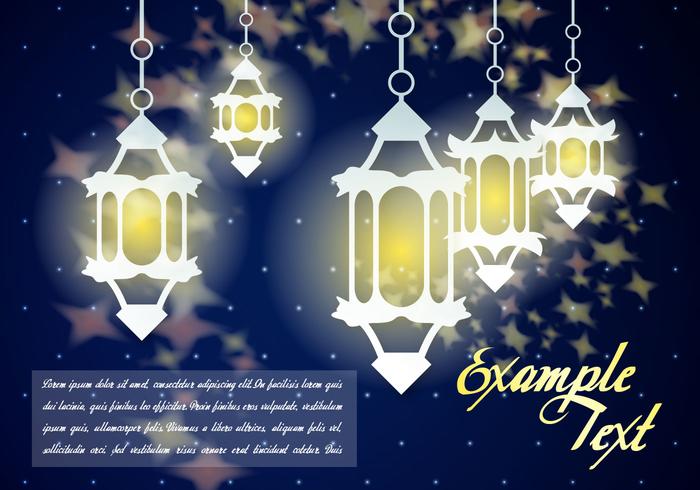The image appears to be a sample graphic, potentially for a greeting card or note card, featuring a dark blue, almost navy background adorned with tiny white dots and faint ghostly images of stars, giving the impression of a starry night sky. The main focus is on the lanterns, which are arranged in two diagonal rows; the larger row extends from the middle right to the upper right, and the smaller row spans from the left to the upper middle left. Each lantern is rectangular with triangular tops and bottoms, and they are white in color, emitting a soft yellowish-orangish glow from within. The lanterns hang from delicate chains illustrated with small circles. In the lower right corner, "example text" is elegantly written in gold cursive, while additional, harder-to-read text appears in small white cursive at the bottom left. This detailed and aesthetically balanced image, with its arranged lanterns and celestial background, could serve well as a customizable template for posters, greeting cards, or advertisements.